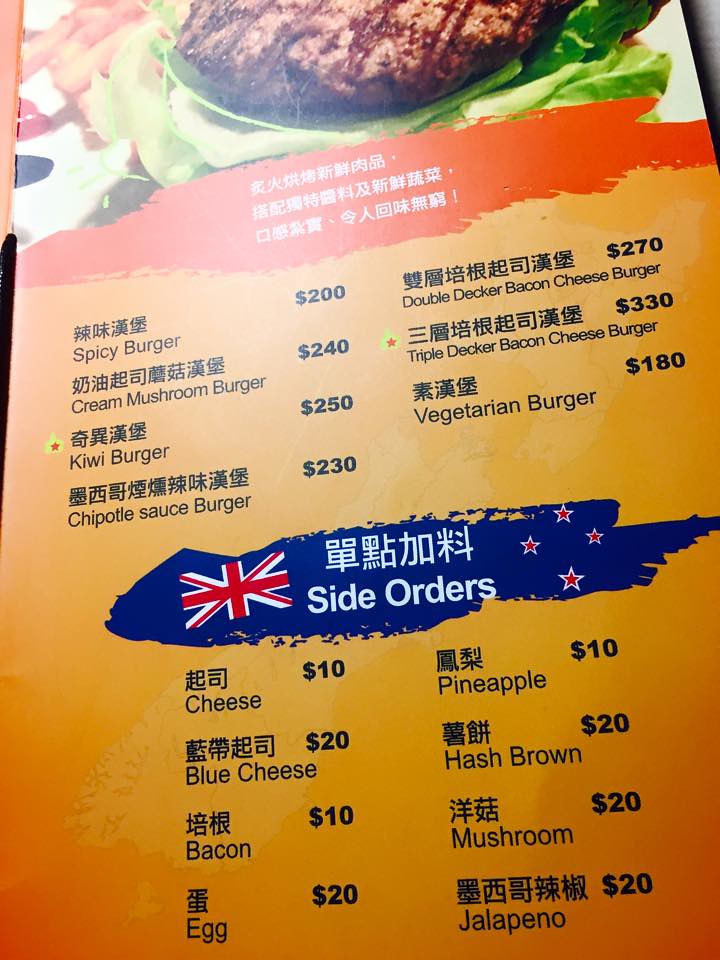Here is a polished and detailed caption for the image described:

"Prominently displayed on a rectangular sheet of paper held lengthwise, the vibrant menu offers a glance into a tantalizing selection of burgers. At the top, a mouthwatering image of a grilled burger nestled on a fresh bed of lettuce captures immediate attention. The menu's background features a gradient, transitioning from a light orange at the top to a rich, darker orange at the bottom.

The menu is bilingual, encompassing both Asian and English text. Listed in dark ink—either a deep blue or black—are the enticing burger options: Spicy Burger priced at $200, Cream Mushroom Burger at $240, Kiwi Burger at $250, and Chipotle Sauce Burger at $230. 

The reverse side of the menu opens with the following delectable choices: Double Decker Bacon Cheeseburger for $270, Triple Decker Bacon Cheeseburger for $330, and Vegetarian Burger for a modest $180. Midway down, a section for 'Side Orders' is introduced, creatively styled to resemble a torn British flag. The left side features a British emblem while the right flaunts white-bordered red stars. Side order options include Cheese for $10, Blue Cheese for $20, Bacon for $10, Egg for $20, Pineapple for $10, Hash Brown for $20, Mushroom for $20, and Jalapeño for $20."